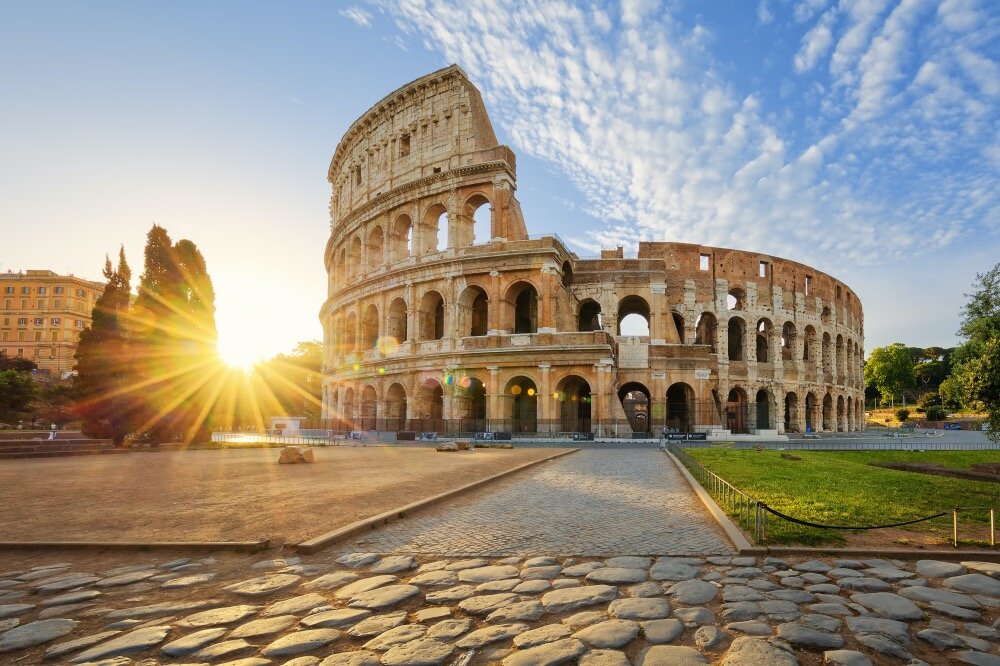This is a detailed exterior view of the ancient Colosseum in Rome, captured under a bright blue sky with clusters of white, high-altitude cirrus clouds. The colossal structure, made of tan stone, features four stories in height but has partially deteriorated over time, with the top two stories missing sections. The lower two floors, however, remain largely intact, showcasing a continuous series of archways that historically provided access to the interior.

To the left of the Colosseum, the scene is bathed in the radiant light of a low-hanging sun, its yellow rays visibly streaming through the sky. The foreground prominently displays a rough, bumpy cobblestone walkway, constructed of large, uneven stones that lead directly to a more refined cement pathway. This smooth path directs the viewer's eyes squarely toward the center entrance of the Colosseum.

On either side of this cement walkway, the ground features contrasting patches of vegetation: a well-maintained expanse of green grass to the right, and a beige, nondescript grassy area to the left, adding textural diversity to the landscape. This composition not only highlights the architectural grandeur of the Colosseum but also encapsulates the historical wear and natural beauty surrounding this iconic monument.